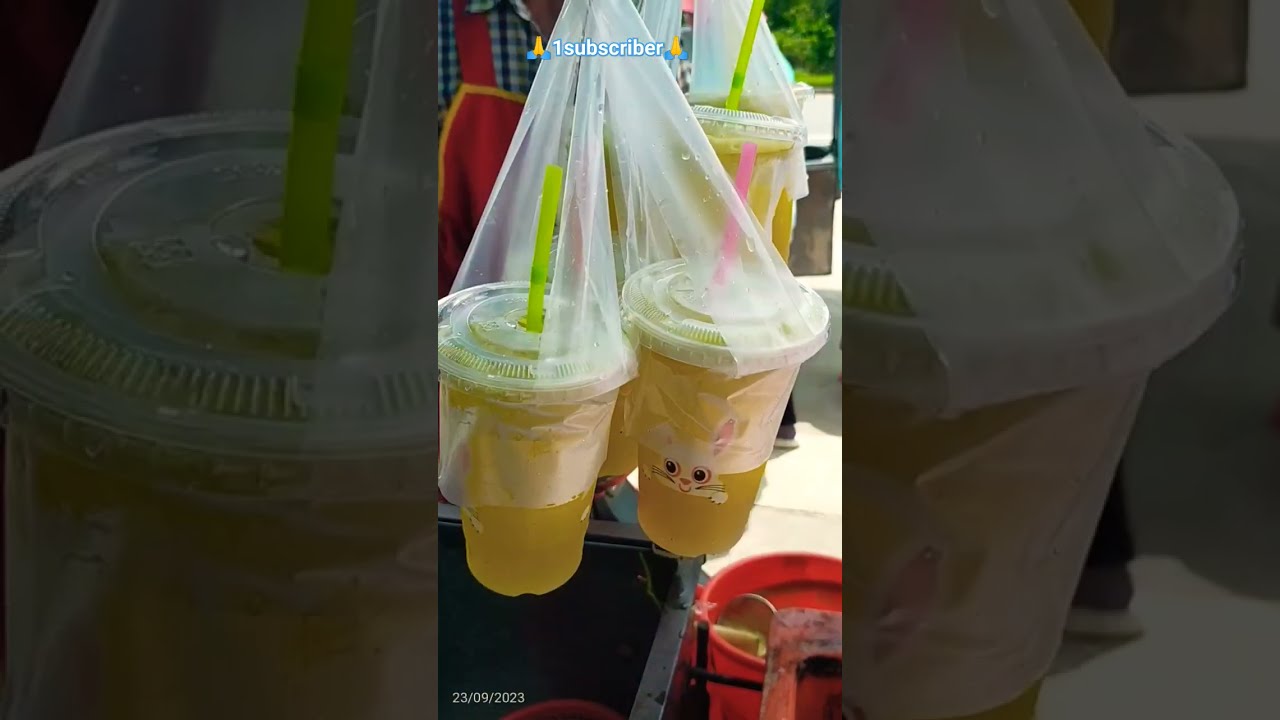This photograph is a horizontally oriented image divided into three panels. The central panel is the main focus, displaying two plastic cups, each with straws emerging from them—one straw is green, the other is pink. These cups, which contain a yellow drink resembling lemonade, are hanging in plastic bags. Above, the plastic bags extend out of the frame, obscuring what they are hanging from. The central panel is the most detailed, showing blurred cups in the background with similar green and pink straws, also hanging in plastic bags. 

The left and right panels are darkened, close-up images of the cups, but they are less clear, creating a faded effect that emphasizes the central panel. The left panel hints at a cup with a yellow straw, while the right panel suggests another cup with a pink straw. In the background of the central panel, additional hanging plastic cups and a blurry tree can be seen. Below the cups, there appears to be a dark object, possibly a stand or a garbage can, partially obscured and difficult to identify. 

Additionally, there is a white text overlay stating "one subscriber" at the top of the central panel, and a date "23-9-2023" on the lower left. The image incorporates a variety of colors including yellow, white, green, pink, blue, red, black, and tan, enhancing the visual complexity of the scene.